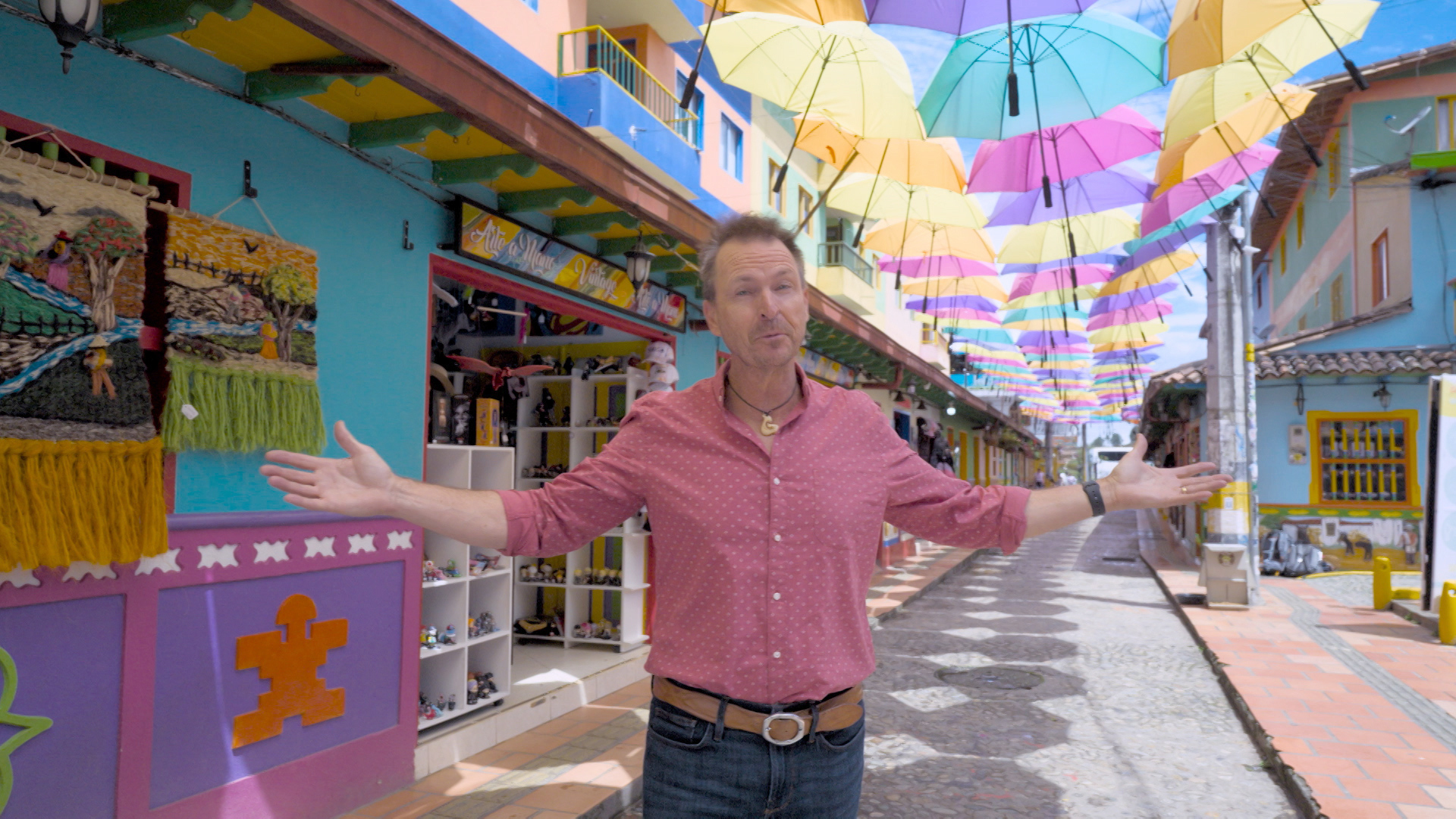In this vibrant and colorful outdoor marketplace scene, an older white man with short gray-brown hair stands prominently in the foreground. He wears a dark pink button-up shirt, sleeves rolled up just below his elbows, blue jeans with a brown belt featuring a silver ring, and a black wristwatch on his right wrist. Around his neck hangs a necklace with a charm. With both arms outstretched and palms up, he appears mid-speech, making a gesture that suggests a shrug. The canopy above him is a striking array of numerous colorful umbrellas, sewn together to cast an intricate shadow over the gray cement walkway beneath. To his left, there are traditional decorations hanging and the entrance to a store, possibly a toy store, is visible with shelves inside. The vibrant street scene, bathed in the midday sun, features light teal-colored buildings with sections of purple, contributing to the lively atmosphere of this bustling outdoor market.